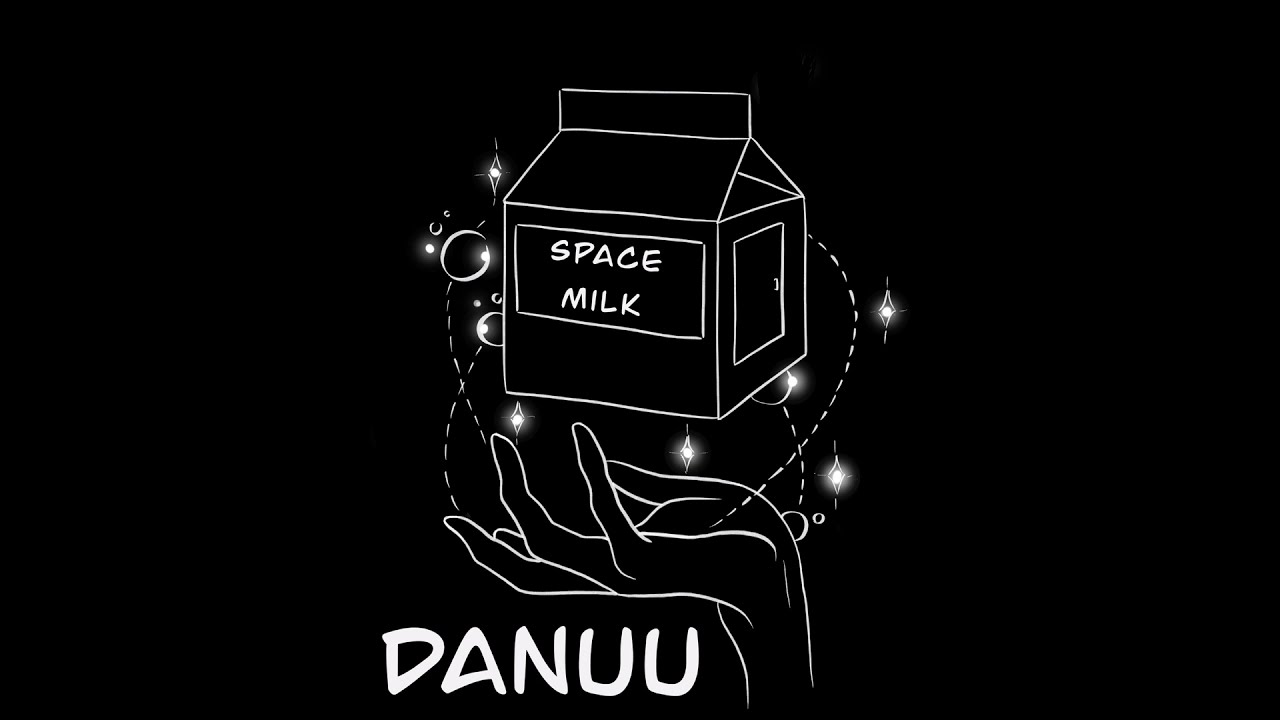In this black and white rectangular image, wider than it is tall, the background is a solid black with intricate white line drawings. Prominently featured in the center is a milk carton designed to resemble a house, which hovers above an outstretched, feminine right hand. The wrist of the hand emerges from the bottom edge of the image, palm facing upwards, back of the hand facing down. Between the hand and the floating carton are orbits of stars and planets, enhancing the space theme with dotted swirling lines and shimmering bubbles and diamonds. The carton itself is angled with one corner towards the viewer. The side facing right has a door, while the front displays a horizontal panel with the text "Space Milk" in bold, cartoonish white font on a black square. Below the hand, at the bottom edge of the image, the text "DANUU" is prominently displayed in all caps, slightly left of the center, completing the artistic and surreal visual.